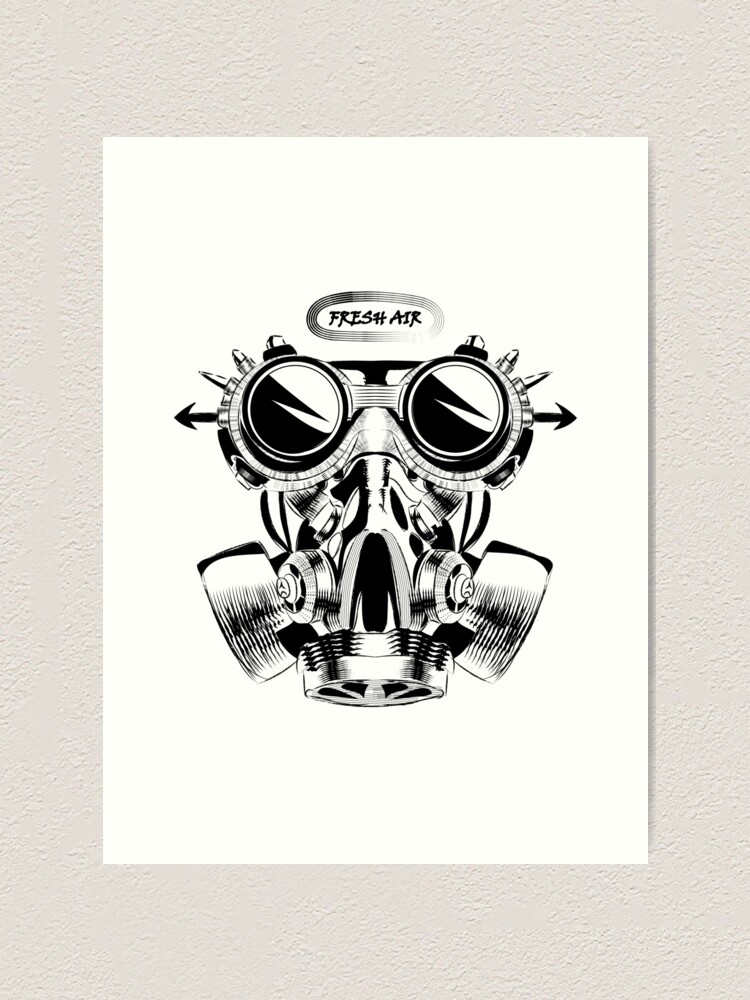The photograph captures a rectangular poster mounted on a textured gray painted wall. The poster itself, also rectangular, features a white background. Dominating the center of the poster is a detailed black and white pencil or pen drawing of a gas mask respirator. This mask has three filters: one on each side of the cheeks and one on the center front. The attached goggles exhibit spikes protruding from the edges, and the lenses are shaded to suggest reflection. Above the gas mask, small handwritten black text reads "fresh air," enclosed in a small five-line oval. The overall illustration has a bold, somewhat futuristic or cyberpunk aesthetic. The image is stark and monochromatic, emphasizing the intricate lines and textures of the gas mask and goggles.